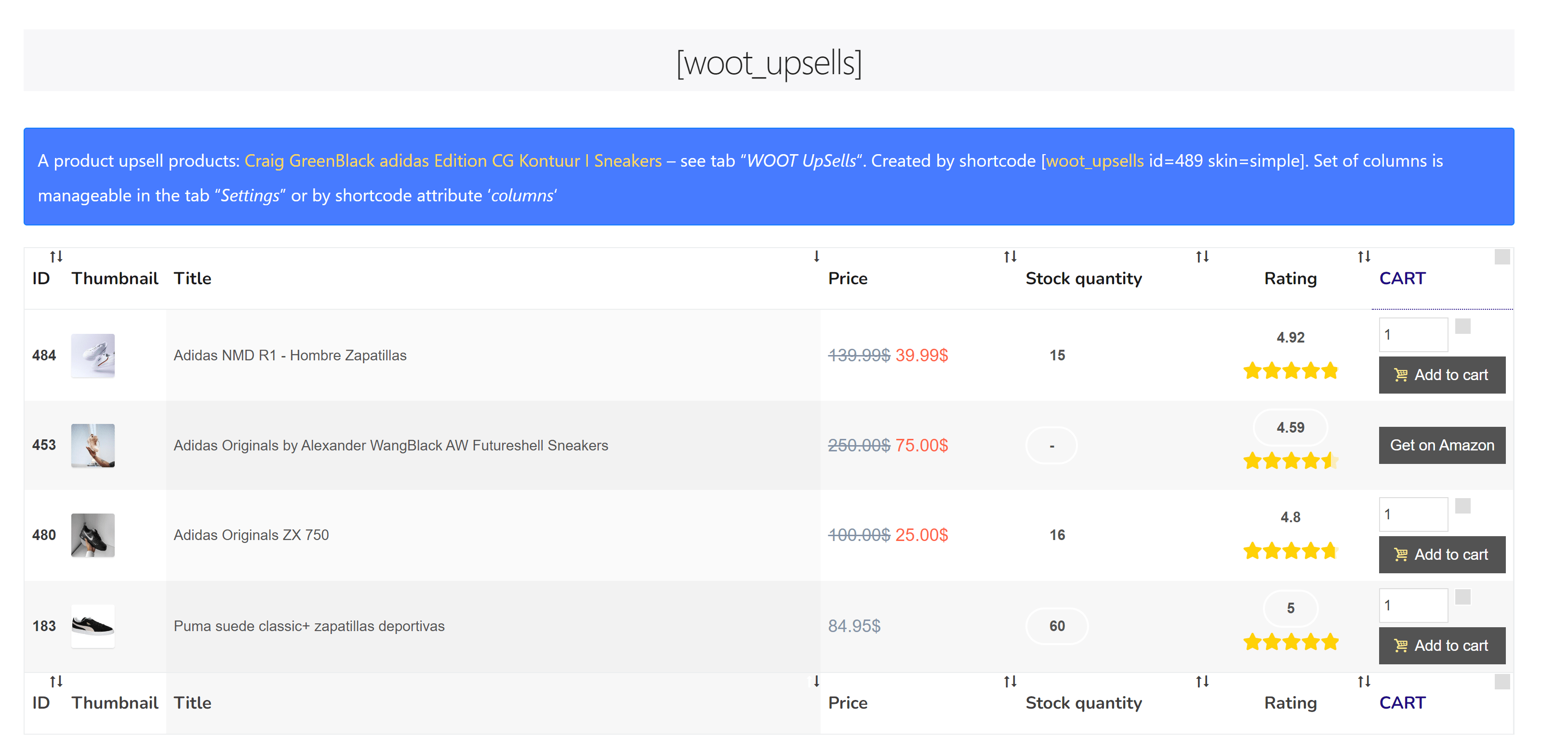The image features a complex chart with various colored rectangles and detailed product information. 

At the top, a light gray rectangle contains the text "[Woot_upsells]". Below it, a blue rectangle labeled "Upsell Products" stands prominently.

Yellow and green rectangles depict product categories:
- Yellow: Craig products
- Green: Black Adidas Edition, CG Contour Sneakers

A white tab labeled "Woot UPSellers" (with "UPSellers" in quotes and "UPS" capitalized) follows. This section is created using a shortcode: [Woot_upsells id=489 skin=simple]. 

Columns are adjustable in this tab through the "columns" attribute in the shortcode. Column headings include:
- ID
- Thumbnail
- Title
- Price
- Stock Quantity
- Rating
- Cart

The first row of data lists:
- ID: 44
- Thumbnail: A small picture
- Title: Adidas NMD R1 Hombres Apitas